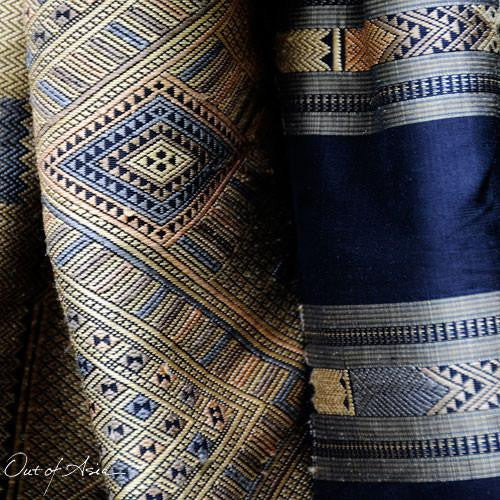The image showcases two intricately woven carpets or cloth pieces. The first piece, on the left, features a diamond-shaped pattern incorporating a subdued palette of blue, green, orangey-red, tan, and faint brown colors. It displays complex designs, including pyramids and winged elements seamlessly woven into the fabric. The second piece, positioned to the right, prominently displays a thick, solid stripe of royal blue alongside alternating light blue and dark blue thinner stripes, each adorned with fine, intricate patterns of pyramids and angular designs. The overall craftsmanship suggests these are handcrafted textiles, possibly featured in a magazine or on a website dedicated to handloom products. A watermark reading "Out of Asia" appears in the bottom left corner of the image.